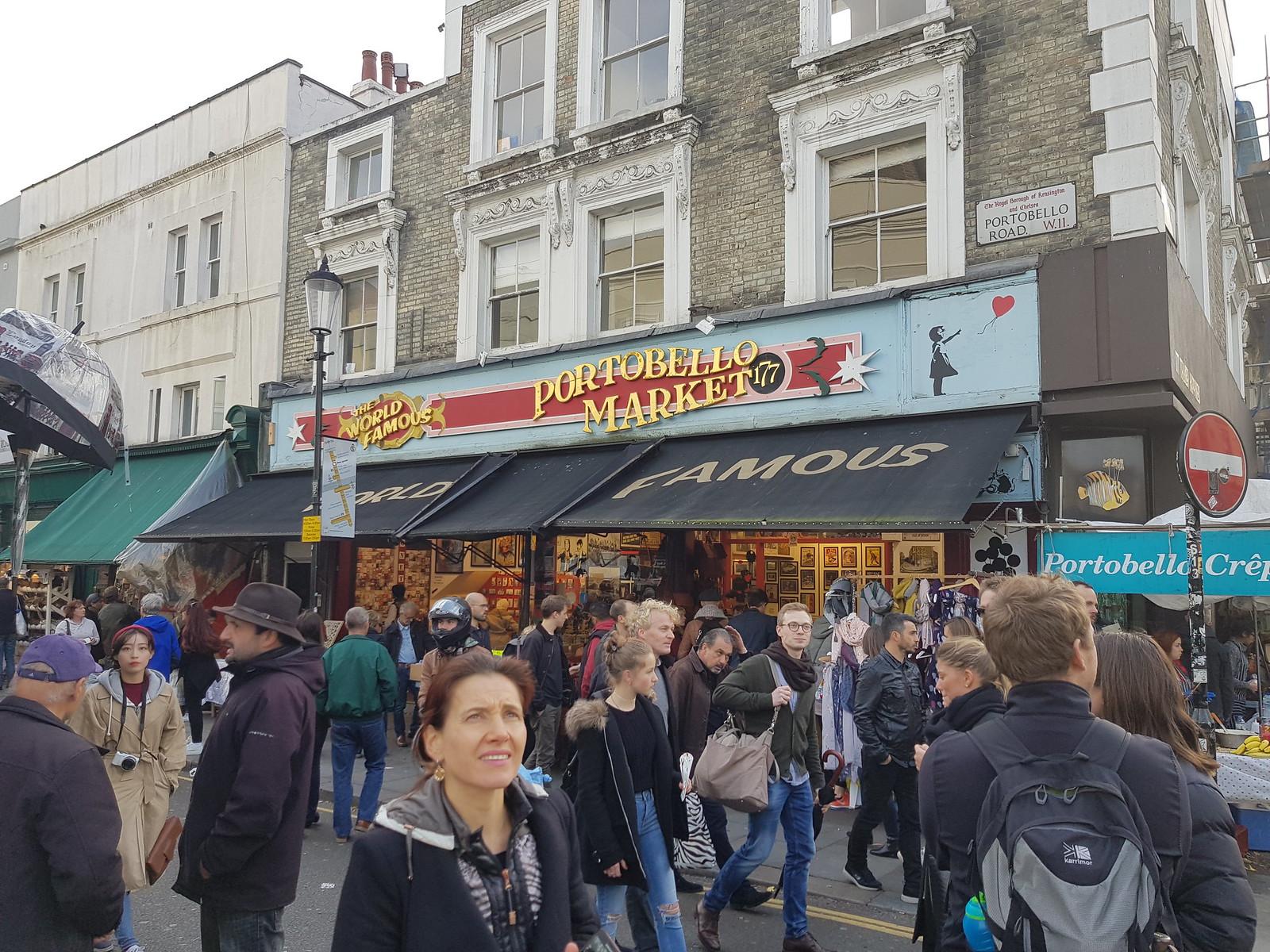This detailed image shows the bustling scene outside the renowned Portobello Market at building 177. The main building is constructed of grayish brick with rectangular windows and prominently displays a sign near the top that reads "Portobello Market" in yellow letters on a red background, with the additional tagline "the world famous" on the left. Another black canopy or awning below also bears the phrase "world famous." The street and sidewalk in front of the building are teeming with people, many of whom are wearing coats. Some individuals are strolling by, while others are casually chatting in small clusters. On the upper right of the building's facade, there is a Banksy graphic depicting the iconic girl with the heart balloon.

Adjacent to this building, in the upper left corner, an older white stone structure with visible streaks can be seen. To the right, another structure houses "Portobello Crepes" and has signage on its second floor that reads "The Royal Borough of Kensington." The street sign on the right confirms the location as "Portobello Road W11," reiterating the area's famous designation.